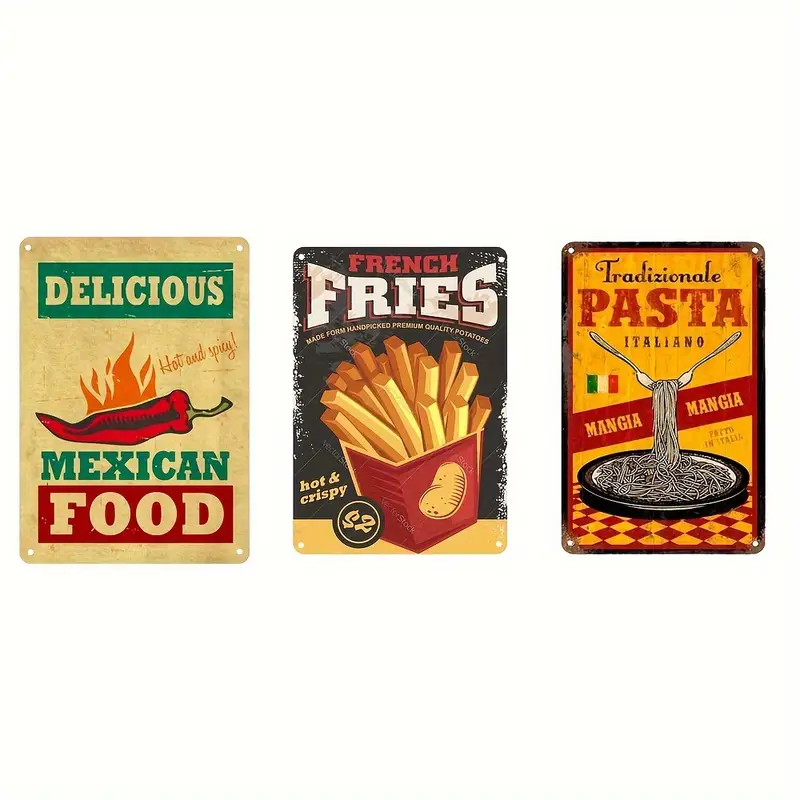This is a series of three vintage food advertisements, likely from the 1950s, each presented on aged metal plates. The first advertisement, with an off-white, weathered background, features the word "delicious" in white on a green block. Below, a red hot chili pepper emits orange flames with the label "hot and spicy." It proudly displays "Mexican food"—"Mexican" in green and "food" in white on a red banner. The second ad depicts a classic promotion for French fries against a black background. A large serving of cartoonish fries in a red container is accompanied by the text "French fries"—"French" in red and "fries" in white. Additional details proclaim the fries as "made from hand-picked premium-quality potatoes," "hot and crispy," and available for "$2" indicated within a black circle. The third advertisement, set against a checkered yellow and red background, highlights "tradizionale pasta Italiano" with "pasta" in bold red and "tradizionale Italiano" in black. Two forks lift a serving of black and white pasta above a plate, with the cheerful "manja manja" (eat up) repeated in a reddish stripe behind. Each plate has visible wear and side holes, suggesting they once adorned the exterior of eateries, encapsulating the nostalgic charm of mid-20th-century food advertising.